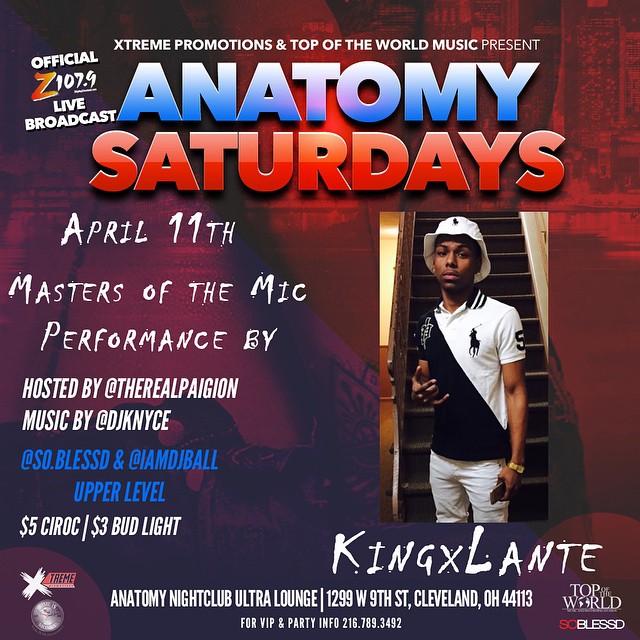This is a highly detailed, computerized promotional flyer for an event titled "Anatomy Saturdays," presented by Extreme Promotions and Top of the World Music. The event features an official Z107.9 live broadcast on April 11th, with a Masters of the Mic performance. The event is hosted by The Real Paggion, with music by DJ KNYCE, DJ So Blessed, and I Am DJ Ball at the Upper Level. The flyer highlights special promotions including $5 Ciroc and $3 Bud Light, and it will be held at Anatomy Nightclub Ultra Lounge, located at 1299 West 9th Street, Cleveland, Ohio, 44113. For VIP and party information, attendees can call 216-789-3492. The background of the flyer includes a red-hued cityscape and various Instagram and Twitter handles are also showcased. On the right side of the image is a photograph of a black man wearing a navy and white polo shirt, white bucket hat, and white pants, holding a cell phone and gesturing with his hand.